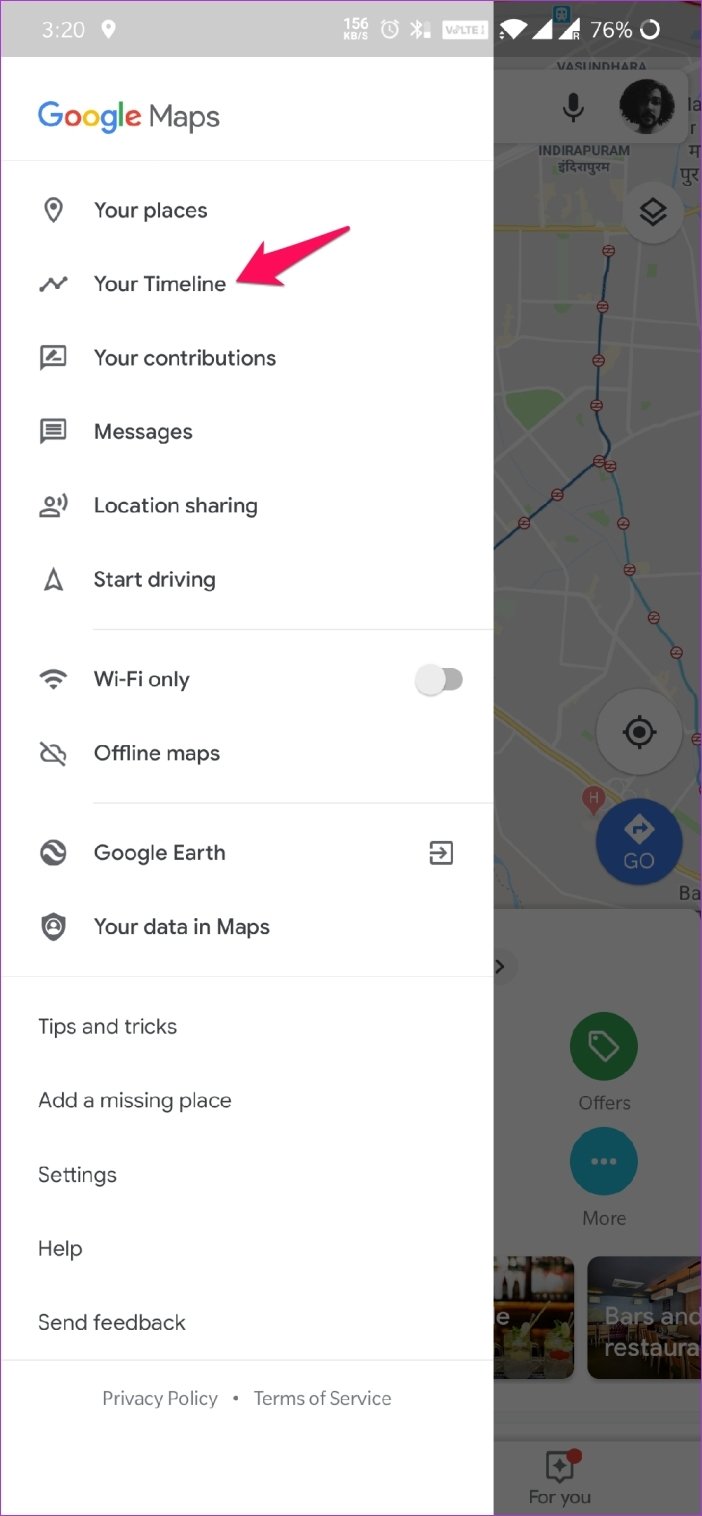The image is a screenshot of a smartphone displaying the Google Maps application. At the top, a dark gray status bar shows white icons indicating the phone's status, including time, battery life, and other essential information.

Covering the left two-thirds of the screen is an elongated vertical menu, presented in a white rectangular overlay. At the top of this menu, "Google Maps" is displayed in text, with "Google" in its distinctive multicolored branding.

The menu lists several options, each accompanied by a black icon on the left:
1. **Your places**
2. **Your timeline**
3. **Your contributions**
4. **Messages**
5. **Location sharing**
6. **Start driving**
7. **Wi-Fi only** - This option includes a toggle switch on the right.
8. **Offline maps**
9. **Google Earth** - This option features a square icon with a right-pointing arrow on the right side.
10. **Your data in Maps**

Following this primary list, there is a secondary list with no accompanying icons:
1. **Tips and tricks**
2. **Add a missing place**
3. **Settings**
4. **Help**
5. **Feedback**

At the very bottom of the menu, separated by a light gray horizontal line, there is a centered gray text stating "Privacy policy • Terms of service," with a dot separating the two phrases.